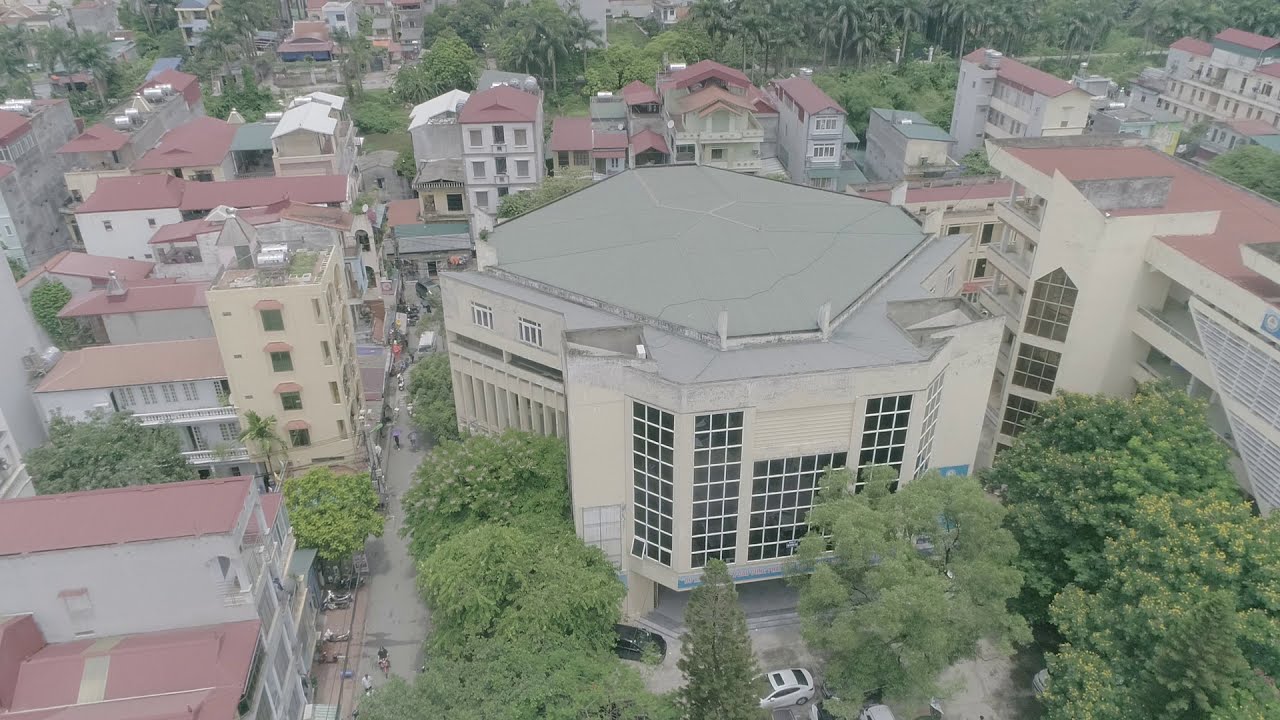This aerial photograph captures a bustling cityscape dominated by a unique seven-sided, concrete building with numerous windows, estimated to be at least 16 stories tall. This central structure, which appears almost circular yet distinctly heptagonal, features a gray, oval-shaped roof. Surrounding this main building are tree-lined landscapes, interspersed with five-story residential homes distinguished by their tan facades and reddish-brown roofs. Palm trees can be seen dotting the background of these residential areas, adding a tropical touch. The image reveals a vibrant and busy environment, with people and cars populating the streets and parking areas. The clarity of a sunny day enhances the overall scene, highlighting the mix of nature and urban architecture.